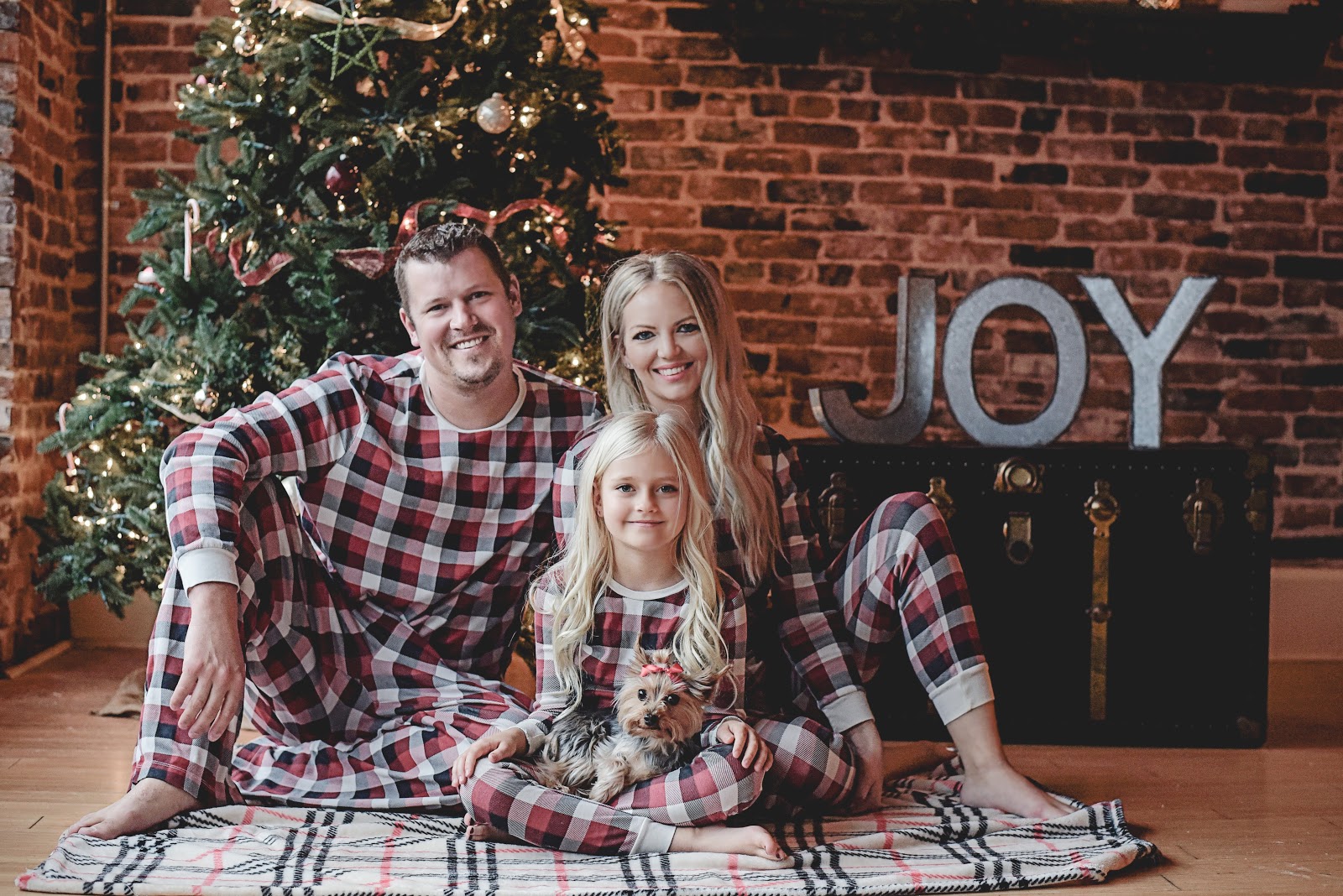In this detailed and warmly festive family portrait, a father, mother, and their young daughter are seated comfortably in front of a beautifully decorated and lit Christmas tree, set against a red brick wall backdrop. The father, positioned directly in front of the tree, sits close to the mother, who is to his right, both wearing matching beige long john pajamas adorned with red and black plaid squares. Their daughter, perched happily between them on a plaid blanket spread out on a wooden floor, crisscrosses her legs and smiles brightly, holding a small dog adorned with a bow in her lap. Behind the mother, a trunk with gold fastenings supports large, silver letters spelling "JOY," adding a touch of holiday cheer to the scene. The setting, likely a photography studio, captures the family in a cozy and joyful holiday moment perfect for their Christmas cards, despite the father's somewhat forced smile.